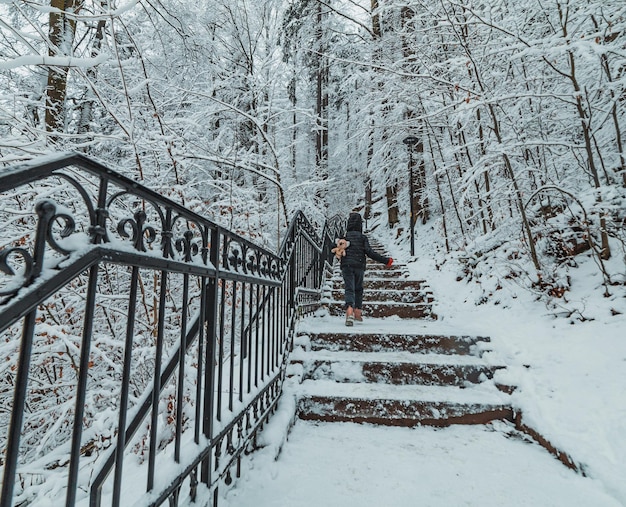This image captures a serene winter scene in a snow-covered forest. Dominating the background are towering trees, each one heavily laden with snow and ice, encasing every branch in a white frost. A stone stairway, blanketed in snow, ascends into this dense, frozen woodland, with a black wrought iron railing flanking its left side. We observe the scene from the base of the steps, where a younger person, clad in a black jacket, black snow pants, red gloves, and pink boots, begins their climb. They have a small, pink backpack or stuffed animal with white ears slung over their shoulder, adding a touch of color to the monochromatic setting. The snowy stairs disappear into the wintry forest, shrouded in an air of mystery and quietude.